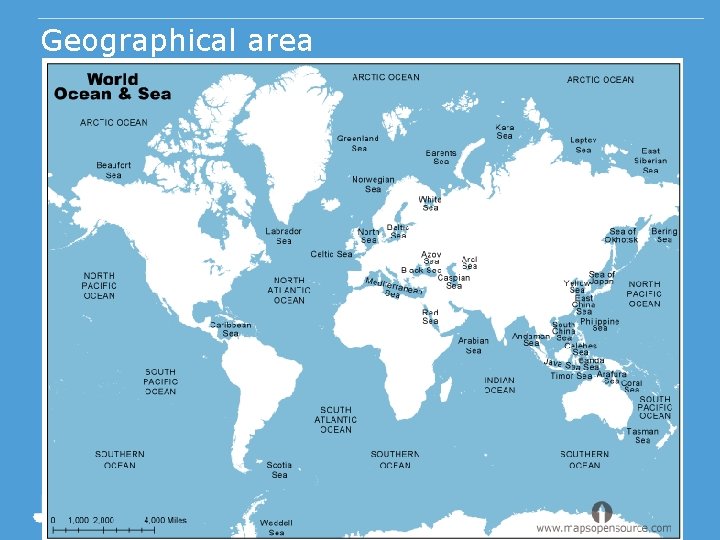The image depicts a detailed graphic illustration of a flattened-out world map. At the very top left-hand corner, in large white sans-serif lettering with a white pinstripe overhead, it reads "geographical area." Just below that, the map is titled "world, ocean, and sea" in black text. The continents are outlined in white against a medium blue ocean background, with the various bodies of water labeled, including the Arctic Ocean at the top center and the Southern Ocean at the bottom center. Also prominently featured are the North Pacific Ocean on the left and right center portions, and other named seas such as the Labrador Sea, Arabian Sea, and Norwegian Sea scattered across the map. The continents appear in white, clearly distinguished from the blue oceans, which are labeled in black. A small logo with the URL www.rrapsopensource.com is located in the bottom right corner, and the entire map is encased in a distinctive white border.